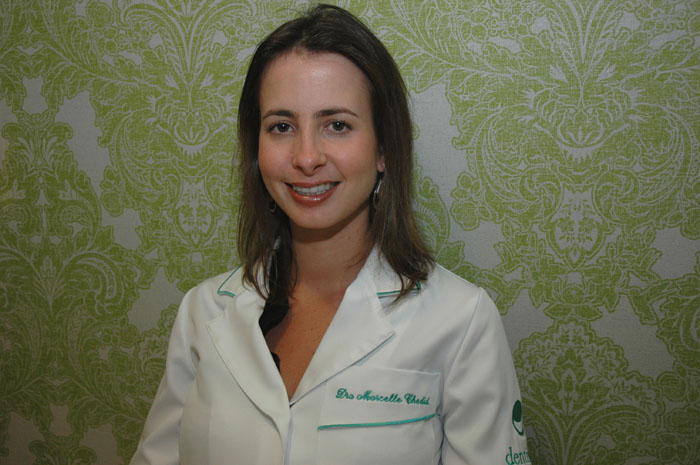This is a detailed portrait of a young woman with shoulder-length brown hair and shiny lip gloss, standing in front of a wall adorned with intricate green and white floral wallpaper, which gives the image an older style appearance. She has pale skin, brown eyes, and is smiling at the camera, revealing her perfect teeth and wearing two looping earrings. She is dressed in a white jacket with teal stitching, which has the embroidery "DEN" visible on her left sleeve, suggesting she may be a dentist. Her name is also embroidered on the left breast of the jacket, but the text is not clearly legible. The photograph is centered on her, showing her from the chest up, and has a slightly darker and professional tone, implying it could be a portrait taken to represent her professional role.